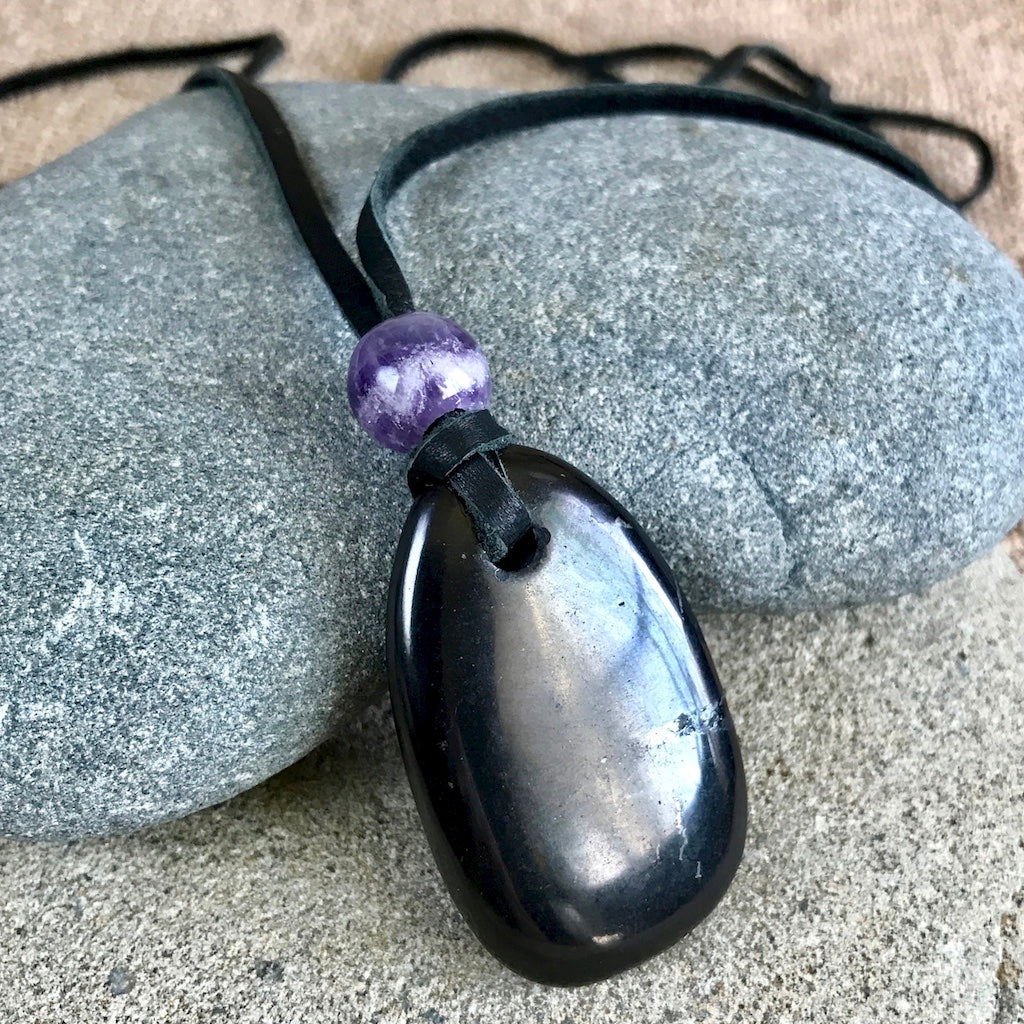The image showcases a detailed close-up of a stone necklace set against a textured background. The main focus is a beautifully shaped gray stone with white flecks, resting prominently on a light sandy-gray, porous rock, possibly soapstone. Central to the image is a heart-shaped gray stone atop the larger gray rock. Atop this heart-shaped stone is a striking black gemstone, rounded at the bottom and resembling a teardrop. This gemstone has a hole punched at the top, through which a black leather band is intricately looped and tied. Just above the knot sits a single purple bead, likely an amethyst, adding a vibrant touch to the composition. The ends of the leather band trail off and disappear behind the gray rock, framing the central elements and adding depth to the composition. The overall bright lighting of the image draws attention to the necklace’s details and the stones' textures, creating a vivid and captivating scene.